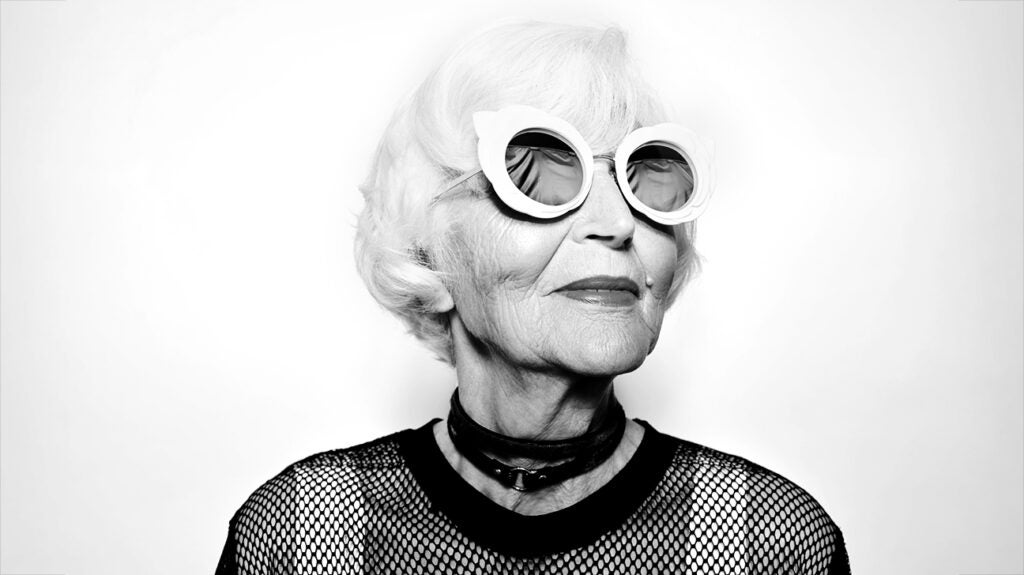In this black-and-white image, an elderly woman with short, white hair styled with bangs appears against a plain, gray backdrop. Her face, marked by a few wrinkles and a distinct mole to the left of her lip, is adorned with lipstick. She wears large, round white sunglasses with a slightly reflective surface, which intriguingly obscure her eyes, creating a distorted view of shapes and skin tones behind the lenses. Her attire includes a layered black choker with a silver clasp at the front and a black fishnet top featuring a thicker black collar and visible straps underneath. The fishnet fabric extends over her shoulders but not below them. This unique combination of elements—her youthful fashion, striking accessories, and the mystery behind her glasses—makes her an intriguing and stylish figure.